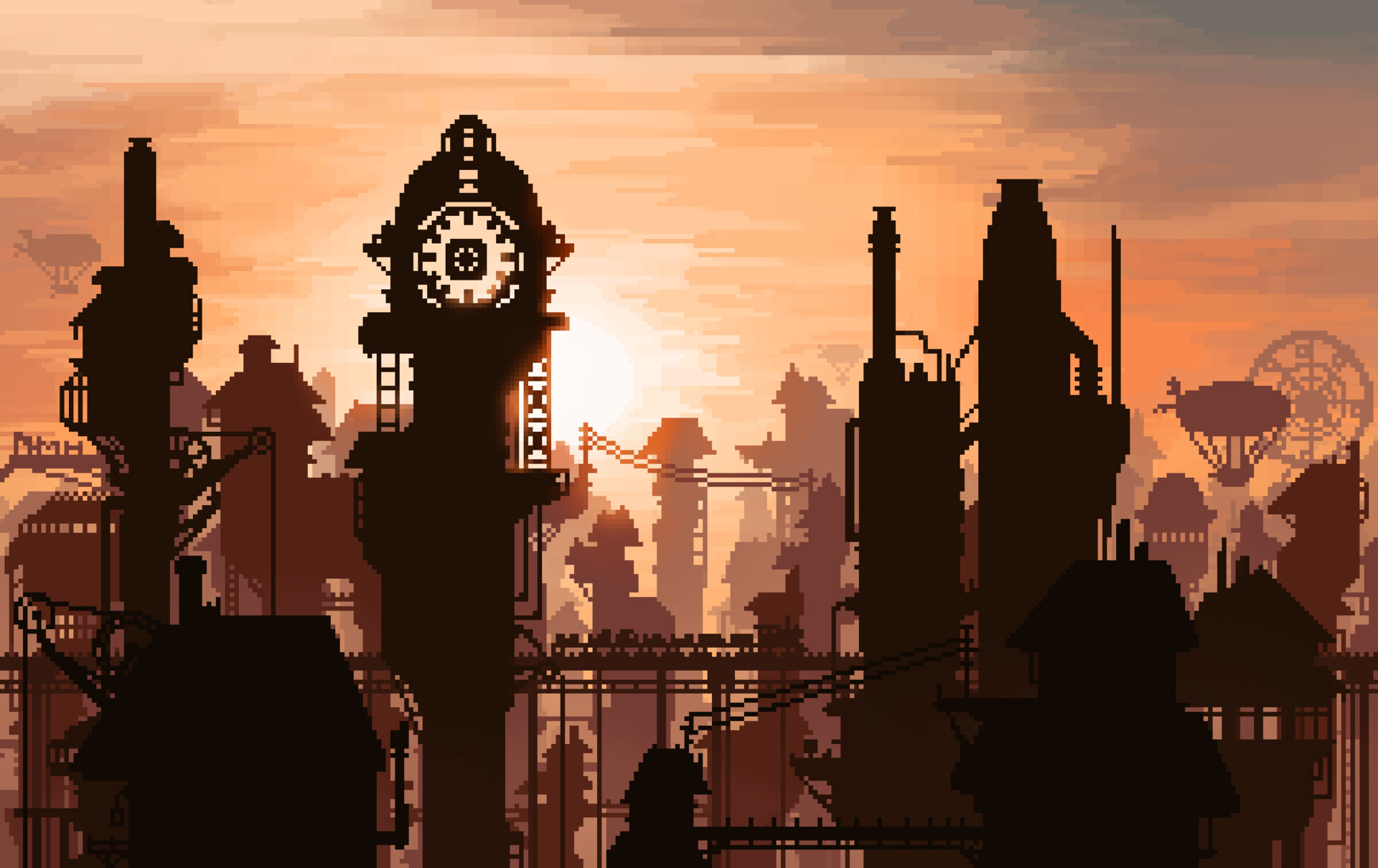The computer-generated image depicts a geometric, futuristic cityscape at sunset, characterized by a pixelated and cartoon-like aesthetic. The sky transitions from vivid oranges and yellows to hints of red and grey, creating an atmospheric backdrop. Silhouetted against this colorful sky are various simplistic yet towering skyscrapers and other industrial-looking buildings, some resembling they are constructed from Legos. 

Prominently featured are several elements that add to the industrial yet whimsical feel: two distinct hot air balloons or Zeppelins on both the right and left sides, and a Ferris wheel situated in the background to the right. Shadows that appear to be human figures are scattered across the foreground. Additionally, a clock tower can be discerned nearby, further enriching the visual narrative of this urban landscape, where the central brightness of the setting sun gradually fades into the darker outskirts of the scene.